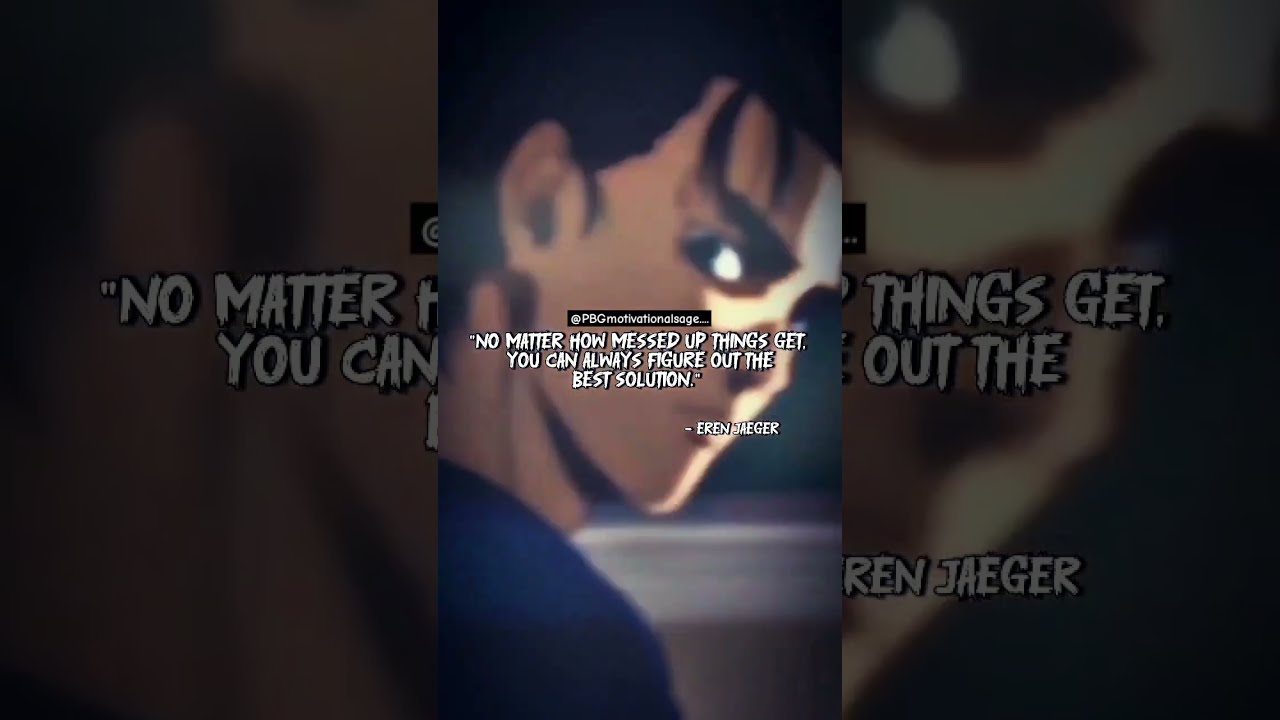The image is a screenshot, possibly from an anime or a video game with anime characters, and seems to mimic the style of a meme. It centers on a cartoon drawing of a young man, likely in his early 20s, with black hair, medium tan complexion, thick black eyebrows, and black eyes. He is wearing a blue shirt and is captured looking slightly over his right shoulder, with two locks of hair falling over his forehead above the outer edge of his right eye. The background features a range of colors including black, tan, white, light blue, dark blue, off-white, and gray. Positioned centrally in the image, both the man's head and the accompanying text are given prominence. The text, written in white lettering, reads, "No matter how messed up things get, you can always figure out the best solution." Below this quote is the name "Eren Yeager," with a black rectangle containing white writing located above the text. Additionally, there is a magnified portion of the same photo on the side, partially showing some of the words. This eloquent setting suggests the image might have been taken from an Instagram post.